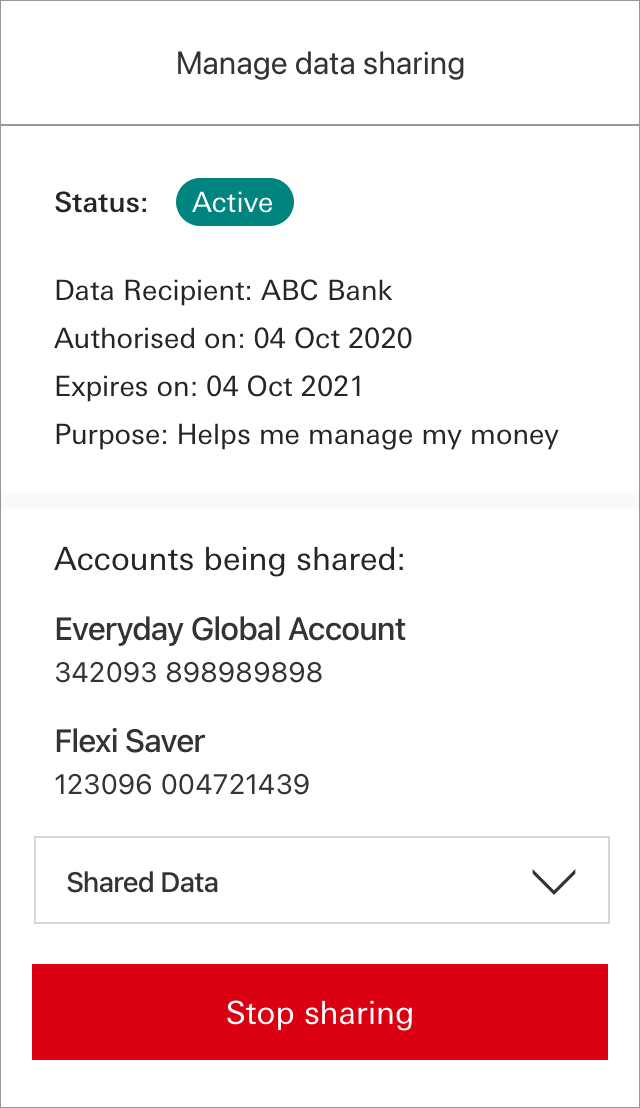This image displays a smartphone webpage designed for managing data sharing permissions. At the top of the webpage, there's a header labeled "Manage Data Sharing."

Below the header, the main body begins with a section titled "Status," which features a prominent green button indicating "Active."

Following the status section, detailed information about the data recipient is provided:
- **Data Recipient:** ABC Bank
- **Authorized On:** October 04, 2020
- **Expires On:** October 04, 2021
- **Purpose:** Helps me manage my money

The next section is devoted to "Accounts Being Shared" and lists:
1. **Everyday Global Account:** Account Number 342093 8989 8989 8989 8
2. **Flex Saver:** Account Number 123096 004721439

Correspondingly, there is a dropdown box under these accounts labeled "Shared Data," which presumably lists the specific data being shared.

At the bottom of the webpage, there is a conspicuous red "Stop Sharing" button that allows the user to terminate data sharing at any time.

The overall status of the page suggests that data sharing is currently active, but users have the control to stop it whenever they deem necessary.